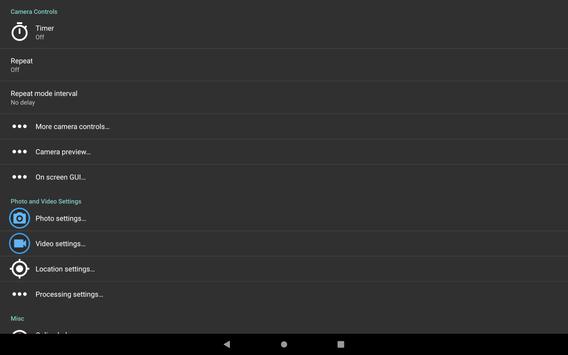Screenshot of an App Interface for Camera Control: 

The screenshot displays a predominantly black screen showcasing an app interface dedicated to camera controls. At the very top of the screen, the title "Camera Controls" is prominently displayed. Below this title, there are two settings: "Timer Off" and "Repeat Off." Following these, there's a section labeled "Repeat Mode Interval," which is currently configured to "No Delay."

Further down, a list of various settings is shown. The settings include options for "More Camera Controls," "Camera Preview," and "On-Screen GUR." The interface also features categories for "Photo and Video Settings," "Location Settings," and "Processing Settings." However, the screen cuts off, preventing visibility of any additional settings that may be listed further down.